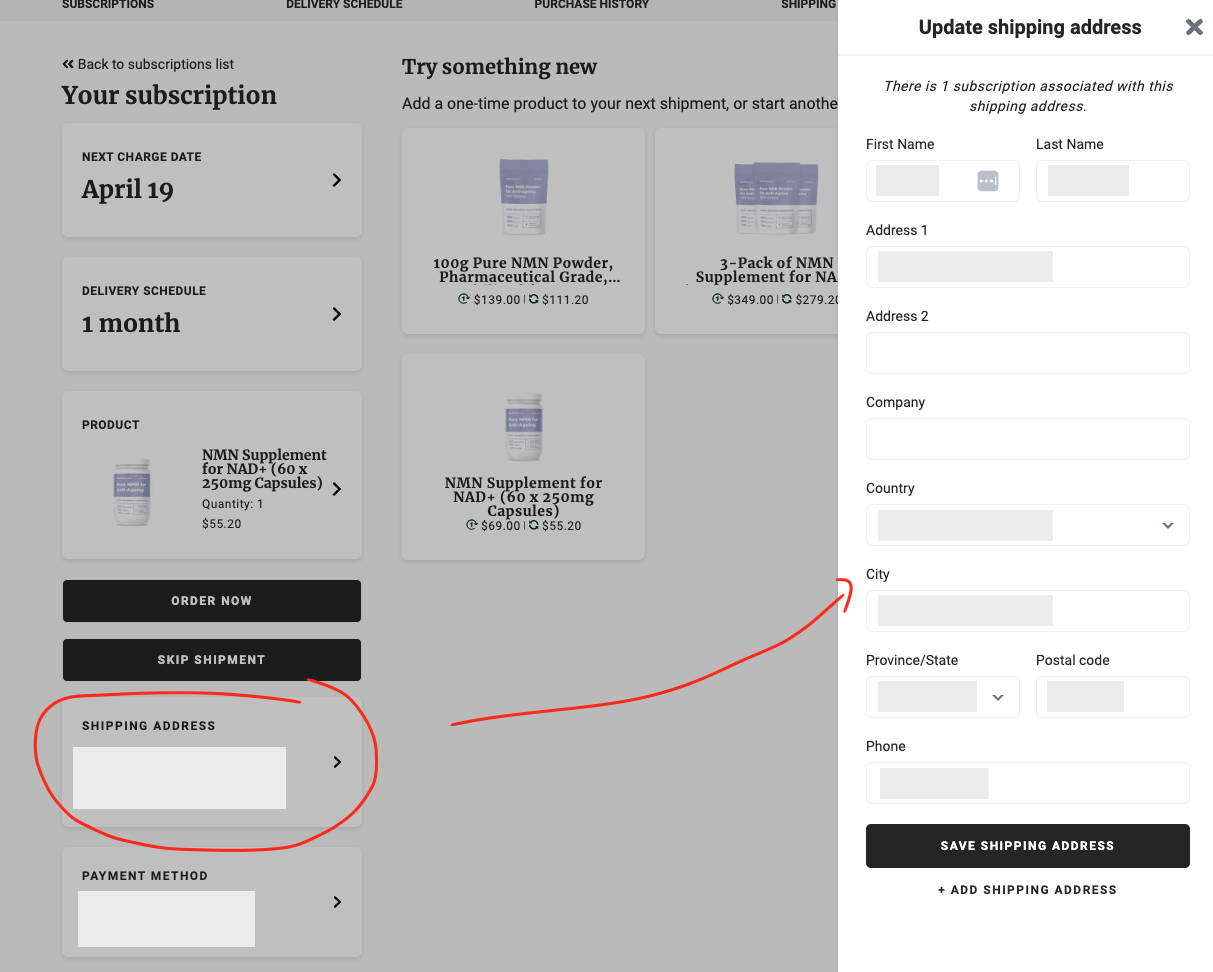Screenshot of a Subscription Management Page for NMN Supplement

The image showcases a detailed screenshot of a subscription management page, primarily focusing on options to update the shipping address. On the left side, the user's subscription details are displayed with navigational arrows. An arrow pointing left, accompanied by the text "Back to Subscriptions List," allows users to return to the main list of subscriptions. Below this, the text "Your Subscription - April 19th" is shown with an arrow pointing to the right, while another arrow directs the user to the right for the "Delivery Schedule - One Month."

The product information section details the subscription product as an NMN supplement for NAD+ with 60 capsules, each 250 mg. The quantity is set at one, priced at $55.20. Below, there are two black buttons labeled "Order Now" and "Skip Shipment," giving users options to manage their order.

The "Shipping Address" section is prominently highlighted and circled in red, indicating its importance. This section contains placeholder text to aid in updating the shipping address, accompanied by an arrow pointing to the right. It also mentions "Payment Method" with placeholder text indicating where users can update their shipping information, clarifying that one subscription is linked to this shipping address.

The form fields for updating shipping details include: First Name, Last Name, Address, Company, Country, City, State, Postal Code, and Phone. At the bottom of this section, a black button labeled "Save Shipping Address" is provided, along with an additional "Add Shipping Address" option below.

Overall, the layout is user-friendly, clearly directing subscribers on how to manage their subscription and update their shipping address efficiently.